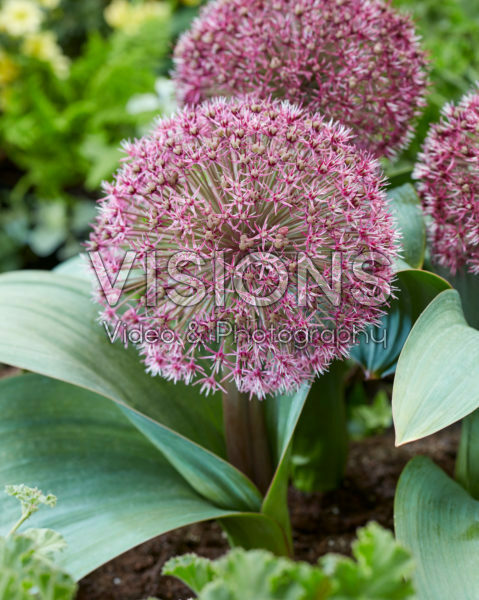This photograph features a close-up view of a plant with a spherical, umbral formation adorned with numerous tiny pink seed heads that resemble a dandelion but are thicker and more densely packed. The plant has a robust, short, and stout stem anchored in rich, dark brown soil. Surrounded by lush, thick green foliage that curves outward, similar to iris leaves, the plant forms a striking contrast against the earthy background. In the foreground, smaller plants peek through, while the background, though out of focus, reveals additional flora, including hints of yellow flowers on the top left and possibly daisies with their signature white petals and yellow centers. This image, devoid of borders and approximately five inches by seven inches in size, also features an overlay of text in the center reading "visions video and photography," indicating a possible digital enhancement. The intricate details and vibrant colors make it a captivating portrayal of diverse plant life in a natural setting.